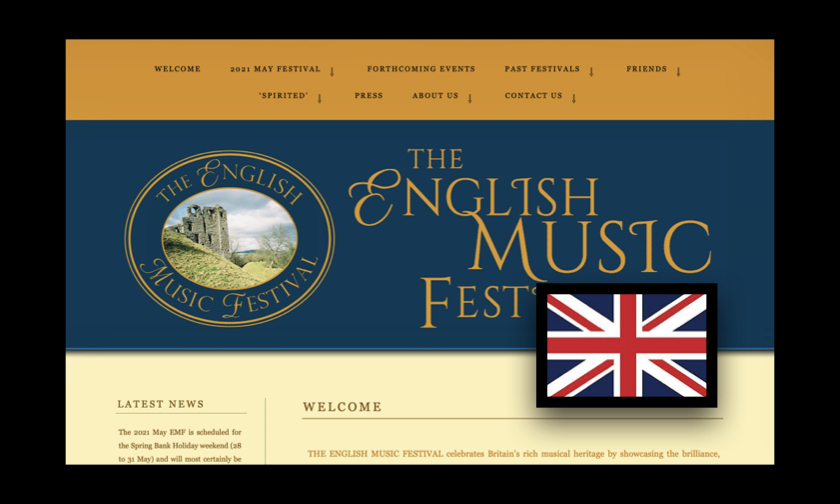This is a detailed screenshot of the English Music Festival's webpage. The layout is rectangular and horizontally oriented with a black border surrounding the contents. The page is divided into three distinct horizontal sections.

The top section has a rich brown background and contains navigation links: "2021," "May," "Forthcoming Events," "Past Events," and "Friends."

The central section stands out with its blue background. On the left side, there is an oval-shaped emblem featuring the words "The English Music Festival" encircling an image of a classic castle. To the right of the emblem, the title "The English Music Fest" is displayed prominently. The latter part of the word "Festival" is overlain by a black-bordered rectangular British flag, adding a patriotic touch.

The bottom section, set against a light yellow, almost beige background, is divided into two main areas. The left area is designated for the "Latest News," providing recent updates and announcements. The right area features a "Welcome Message" to greet visitors and introduce them to the festival's offerings.

Overall, the design balances text and imagery to create an informative and visually appealing interface.